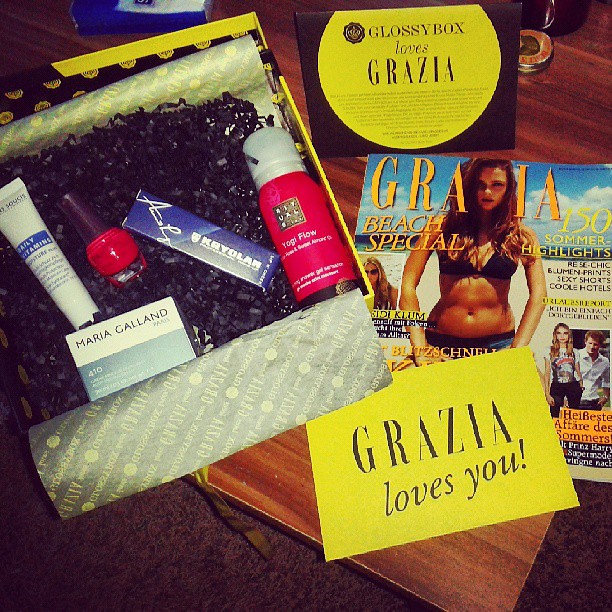The image captures an overhead view of a wooden coffee table adorned with various items. At the center, there's a yellow piece of paper prominently displaying the message "Grazia loves you." Above this paper is a copy of Grazia magazine, featuring a young woman in a bikini on the front cover with headlines like "Beach Special" and "150 Summer Highlights." Just above the magazine is another yellow card stating "Glossy Box loves Grazia," accompanied by additional, smaller text. To the left of the magazine, there is an opened gift box lined with a yellow border, containing five beauty products. These products include a red Yogi Flow item, a Maria Galland daily vitamins lotion bottle, a red lipstick, and two other unspecified beauty items. The table is set against a backdrop of short carpeting.